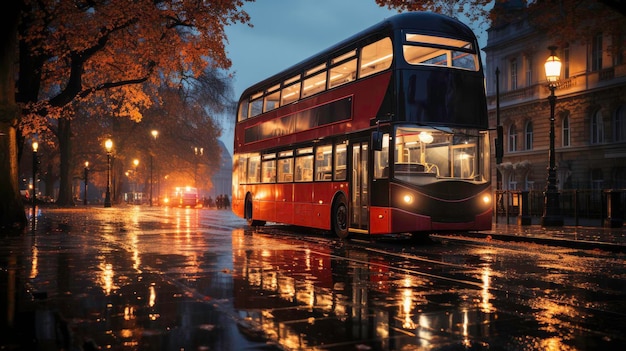This nighttime scene features a red, London-style double-decker bus, likely computer-generated, prominently displayed on a wet road. The bus is oriented towards the right and angled with its closest corner on the right side, revealing its two levels through large windows. The street is illuminated by classic, old-fashioned lampposts and the bus's headlights and interior lights, creating reflections on the rain-soaked pavement. Flanking the bus are a tall street lamp to its left and a brick, three-story building to its upper right. In the backdrop, there's a dark sky peeking through with a mix of trees—possibly oak with red and orange leaves indicative of fall or early winter—and another vehicle and pedestrians walking along the sidewalk that runs between the bus and the buildings.